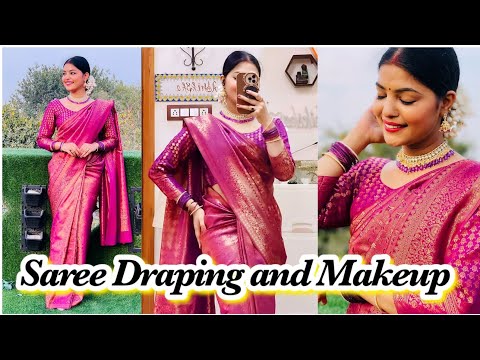The image is a thumbnail, likely for a YouTube video or tutorial, featuring a model shown three times in different poses, with thick black bars at the top and bottom, which are typical of video screenshots. The text on the image, in a bold black font with white backing and glowing yellow edges, reads "Saree Draping and Makeup." The model is adorned in a beautiful fuchsia sari with a blend of purple, pink, and copper hues, accented by a faint golden design of dots and stripes. Her makeup is meticulously done, highlighting her flawless complexion and red lips. 

In the leftmost picture, the woman stands in a lush, green outdoor setting, with trees and shrubbery behind her. Her black hair, adorned with a flower, is elegantly pulled back. She stands gracefully, showcasing her full-length sari. In the middle image, she is indoors, holding a phone up to her face as if taking a selfie, with signs and pictures visible on the walls behind her. The rightmost image is a close-up shot from her head to her stomach, where she stands with closed eyes and a smile, displaying her makeup and jewelry, including several necklaces and bracelets, and a decorative flower or jeweled ornament on her neck.

Overall, the thumbnail gives a comprehensive visual guide on sari draping and makeup, wrapped in a blend of tradition and modern presentation, designed to appeal to young women interested in East Indian fashion and beauty techniques.